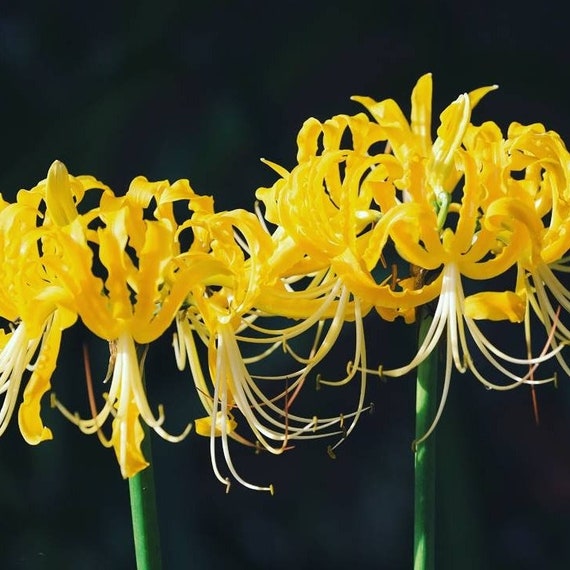The photograph features two partially bloomed yellow flowers positioned against a blurred backdrop of dark green and black hues. The flowers stand with their green stems stretching downward, though cropped at the image's bottom. Their yellow petals appear slightly curled, resembling lemon rinds, which suggests they are either in the early stages of blooming or nearing the end of their life cycle. The flowers' centers, exposed and vulnerable, seem poised to attract pollinators for fertilization. Entwined among the petals are small white elements, possibly undeveloped petals or tiny seeds, adding intricate detail to the scene. The dark, indistinct background accentuates the vibrant colors and delicate structures of the flowers, creating a striking contrast.